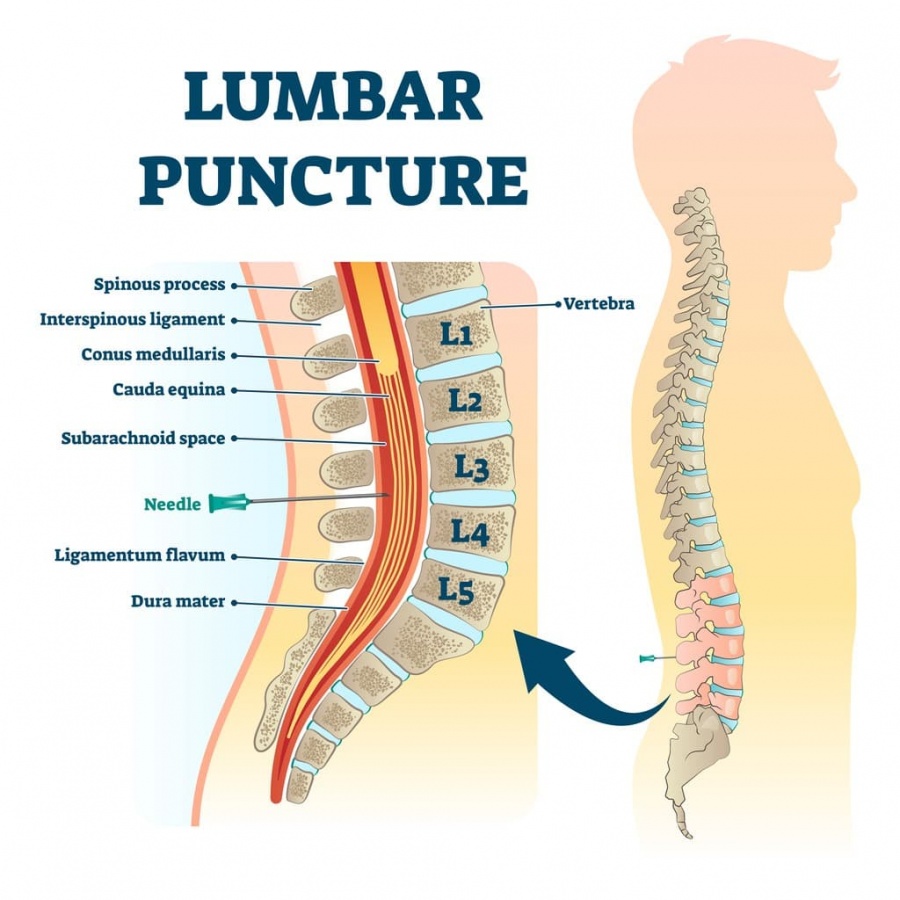This digital image is a detailed medical diagram titled "LUMBAR PUNCTURE," displayed in dark blue capital letters at the top left corner. The background of the image is white. On the right side, there is an outline of a human figure in light pink, within which is a diagram of the spinal cord depicted using light gray, blue, and pink colors. This diagram highlights the lumbar region of the spine, specifically from vertebrae L1 to L5, with an arrow pointing to L5.

To the left side of the human figure, a close-up view of the spinal cord diagram is shown, with various parts labeled in blue. The labels include key anatomical components such as the spinous process, intraspinous ligament, conus medullaris, cauda equina, subarachnoid space, and dura mater. The close-up also indicates the location for a lumbar puncture needle, depicted in green, and the ligamentum flavum.

The diagram uses a range of colors including pale orange, pale yellow, pink, light blue, red, and green, to differentiate between various anatomical structures and to provide clarity in the depiction of the spinal components. This medical diagram is intended to aid in the understanding of a lumbar puncture procedure by providing a detailed illustration of the relevant spinal anatomy.